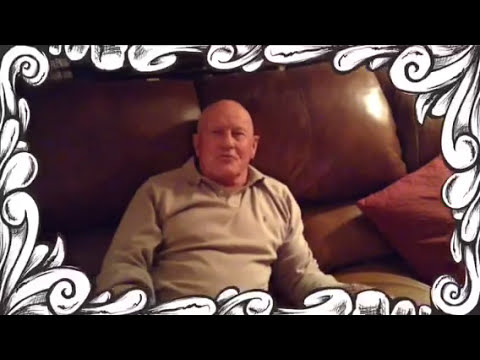The photograph portrays an older, bald man sitting on a brown leather couch with three cushions. A red or burgundy pillow rests in the corner to his right. He is dressed in a somewhat wrinkled tan long-sleeve button-down shirt. He appears to be in his 50s or 60s and is slouched slightly, his left elbow resting on the couch cushion. His expression is somewhat ambiguous; his pursed lips suggest he might be about to speak, and his eyes are only partially open as he faces forward. The image is framed by a black horizontal stripe at the top and bottom, and within that, a decorative white border with black outlines, featuring flowery, swirly, leaf-like patterns.